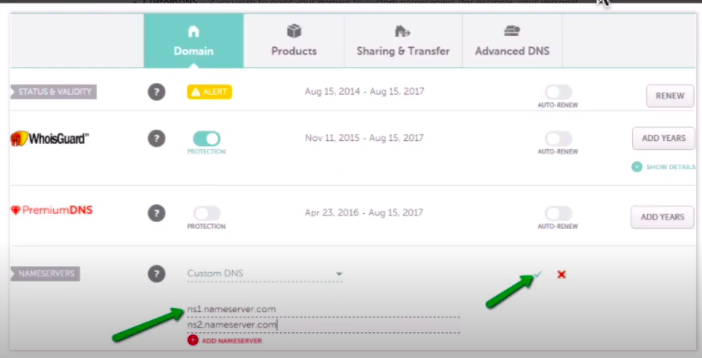The image displays an interface related to domain management, with detailed sections for product, shipping, and transfer information. Prominently, advanced DNS settings and their status and validity are showcased. The image features “HolGuard Premium DNS” with question marks beside each entry. Dates highlighted include August 15, 2014, and August 15, 2017. Options for toggling auto-renew and renewing the service are visible, with additional controls for enabling protection between November 11, 2015, and August 15, 2017. Another toggle for adding years to the service duration is visible, accompanied by a “Toggle Nutrition” button, specifying a range from April 23, 2016, to August 15, 2017. A green arrow points to "assembler1nameserver.com" and another to a green checkmark next to a red X. The bottom right corner of the interface has a white background.